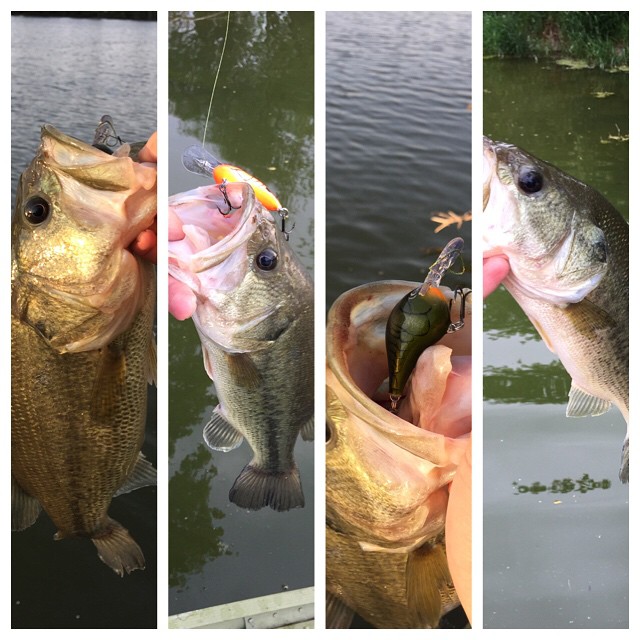This square, color photograph is divided into four vertical portrait-mode images, each separated by white lines, collectively depicting the capture of a medium-sized bass in vivid detail. Moving from left to right:

1. The first image shows a dark green, gray-finned bass with its mouth held open by a visible right hand, against a backdrop of water.
2. The second image reveals the same bass, now featuring a yellow lure still lodged in its mouth, with the water behind it.
3. The third image offers a downward perspective into the open mouth of the bass, showcasing the yellow lure in clearer detail and the greenish tone of the water.
4. The fourth and final image presents another close-up of the bass, displaying its black eye, light gray body with a white underside, set against the water's dark hue.

In all photos, the fish is the centerpiece, with its freshly caught state highlighted by the lure and the natural aquatic environment.